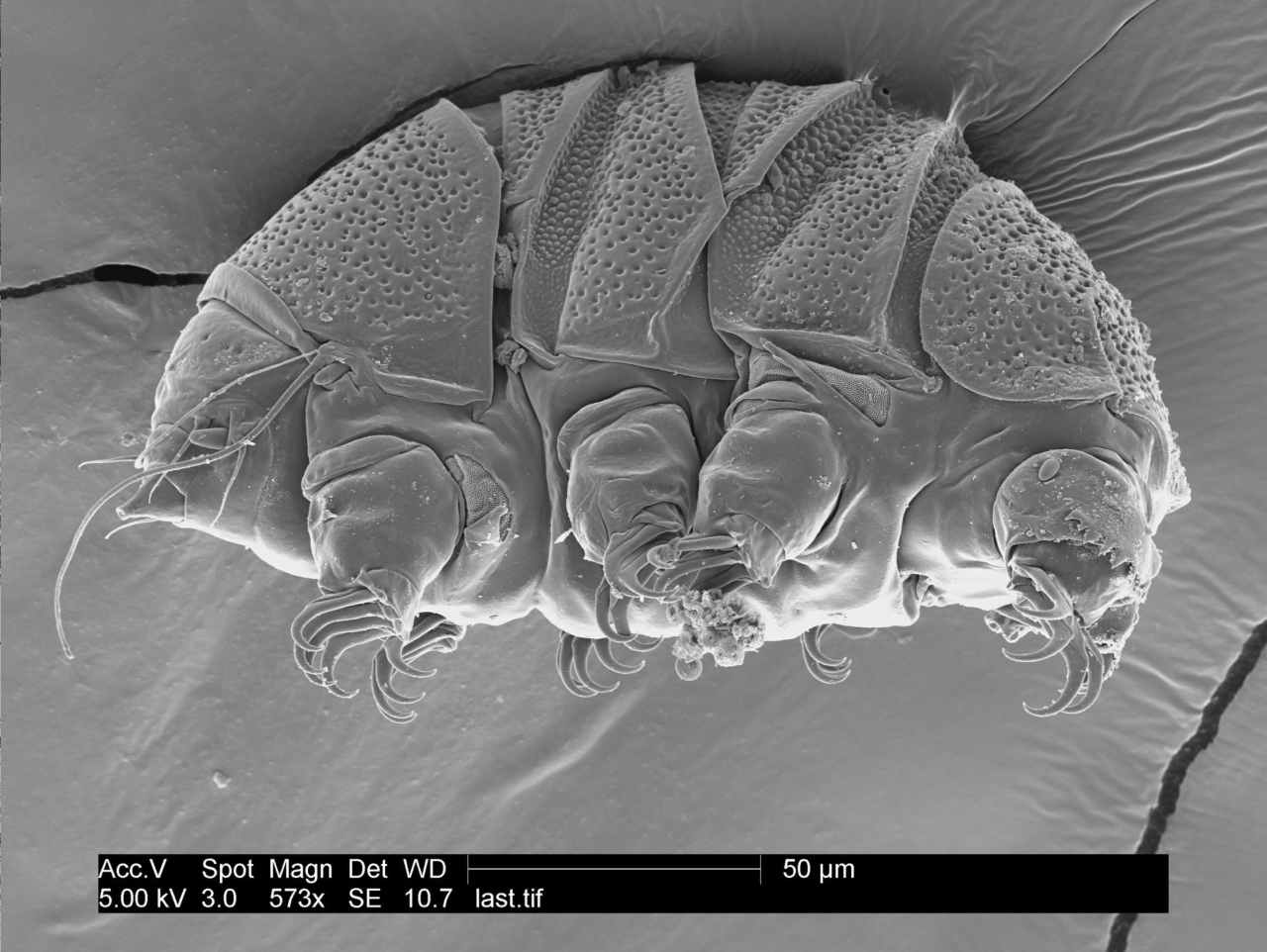The image showcases a highly magnified view (573x) that appears to be of a microscopic organism, resembling a tardigrade, detailed in shades of gray and white. The creature features eight segmented, white legs and a pointed mouth area, reminiscent of an anteater's snout. Its exterior is textured, somewhat leathery and armor-like, with numerous pockmarks. At the bottom of the image, there is a black strip with white text displaying various details, including "ACC.V," "SPA 3.0," "5KV," "573X," "DET SE," "WD 10.7," "LAST.TIF," and "50 µm," indicating specific data related to the magnification and imaging conditions. The gathered material appearance, as previously likened to a satin evening bag, contributes to the textured and intricate portrayal of the microscopic subject.